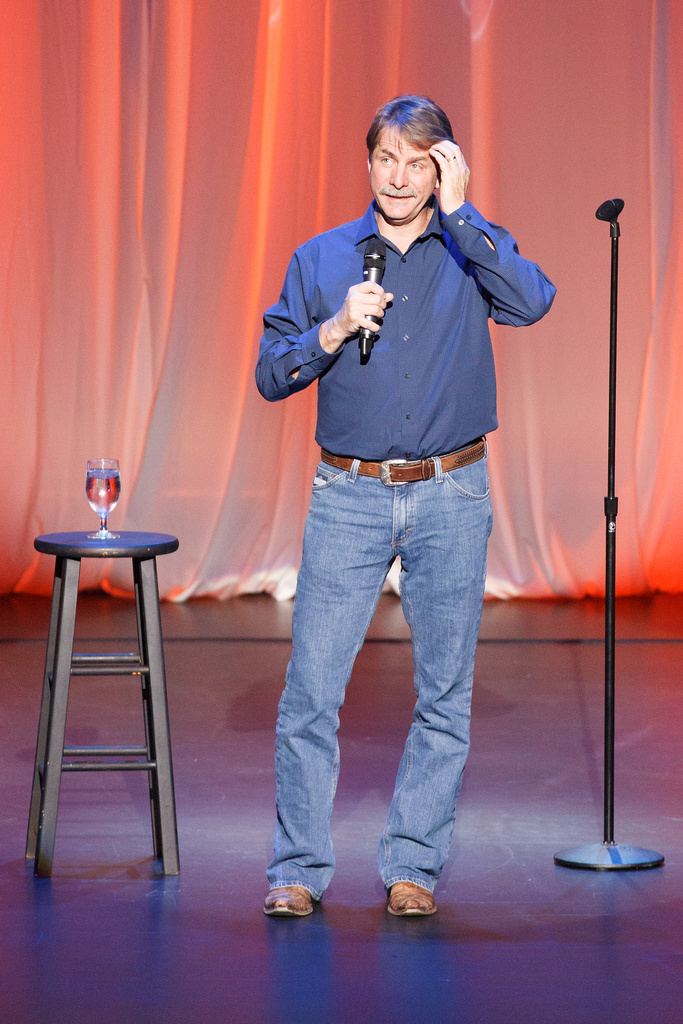In this image, we see comedian Jeff Foxworthy standing on a stage with a red curtain backdrop, illuminated by a spotlight. He features a gray mustache and light brown hair that is parted to the side. Jeff is dressed in a dark blue button-down shirt with a collar, which is unbuttoned at the top, paired with blue jeans, a brown belt, and cowboy-esque brown shoes. He holds a wireless black microphone in his right hand, close to his face, and his left hand is scratching the side of his forehead. To his right stands a tall microphone stand with a metal knob for height adjustment, and to his left is a black wooden stool bearing a wine glass filled with a clear liquid, possibly water. White curtains with orange reflections from lighting add depth to the scene, emphasizing the indoor setting likely designed for his performance.